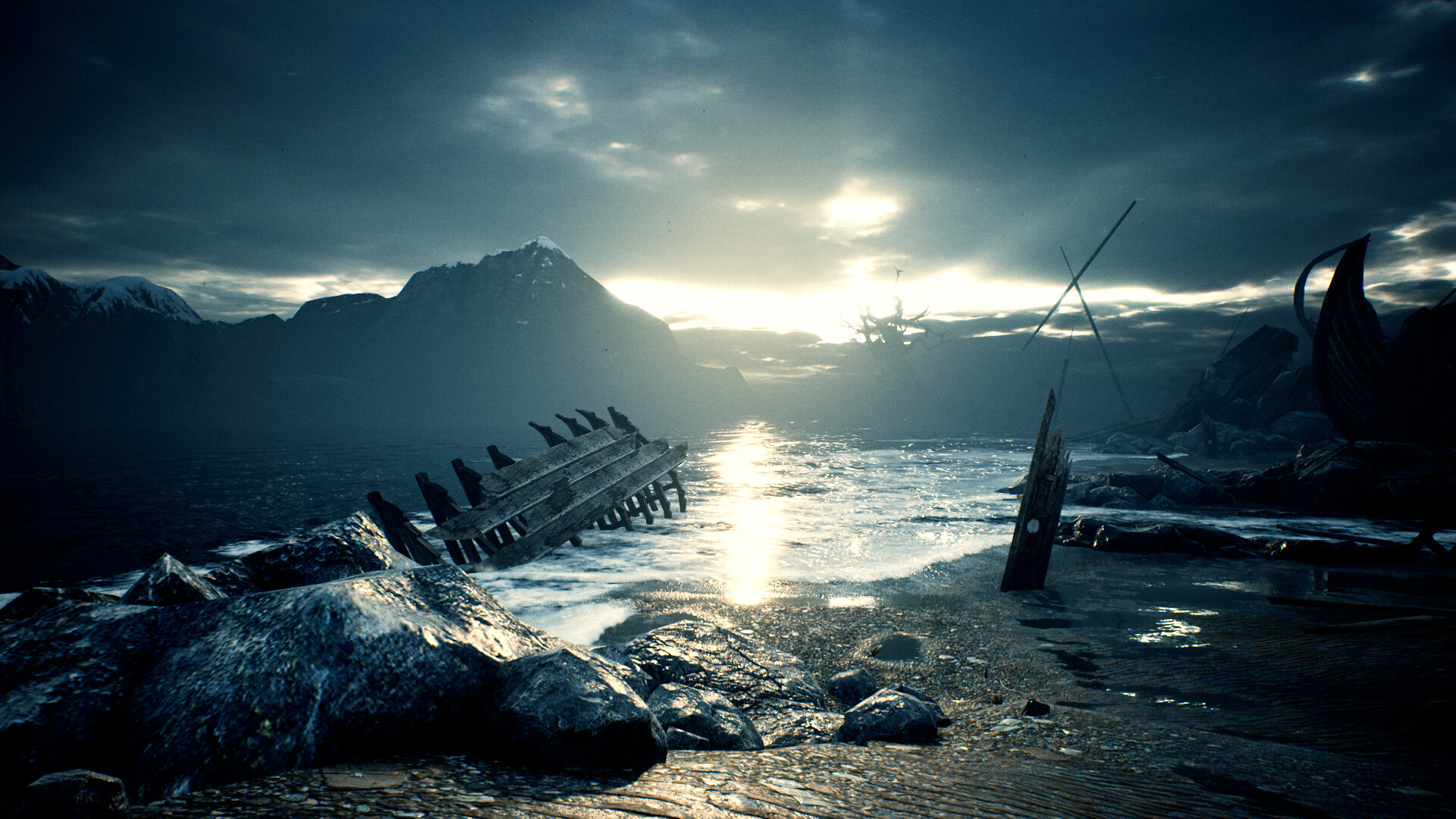This highly detailed and eerily atmospheric image portrays a rocky, desolate beach during what appears to be a hyper-realistic, computer-generated sunset. The focal point of the scene is a series of old shipwrecks scattered across the treacherous coastline, with remnants of broken wooden structures—possibly part of a bridge—adding to the haunting effect. In the background, snow-capped mountains loom under dark grey clouds, while the sun peers through the gaps, casting a reflective glow on the calm yet ominous ocean waters. The texture of the sand, rocks, and scattered leaves is meticulously rendered, evoking the feel of a high-stakes video game environment or a still from a dramatic movie. The overall palette is dominated by dark greys and cold blues, enhancing the scene's ghostly and desolate vibe.